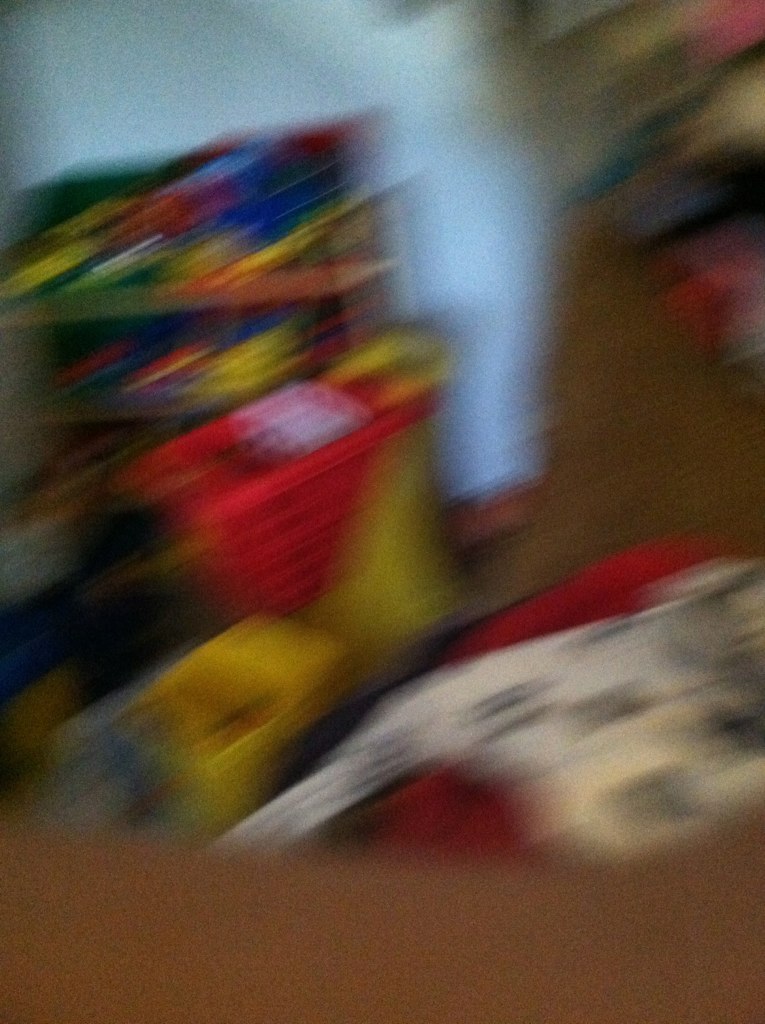This color photograph is very blurry and difficult to discern due to apparent camera movement. The image, rectangular and vertical, appears to capture a children's playroom or classroom. A red plastic shopping cart with a yellow handle is discernible on the left side. Next to it, there seems to be a small yellow toy truck. In the background, a white wall is partially visible, with a shelving unit that holds various brightly colored objects, possibly toys or papers, in hues of yellow, blue, and red. On the right side of the image, there appears to be a red desk with a drawing or image of a dog on top. The bottom sixth of the photo features a brown-colored surface, which might be a wooden or carpeted floor. Additionally, there may be the skin of someone's arm visible at the bottom. The upper right-hand corner of the photo is dark, displaying shades of red, yellow, and yellow-green. The overall blur makes it challenging to pinpoint specific details and objects clearly.